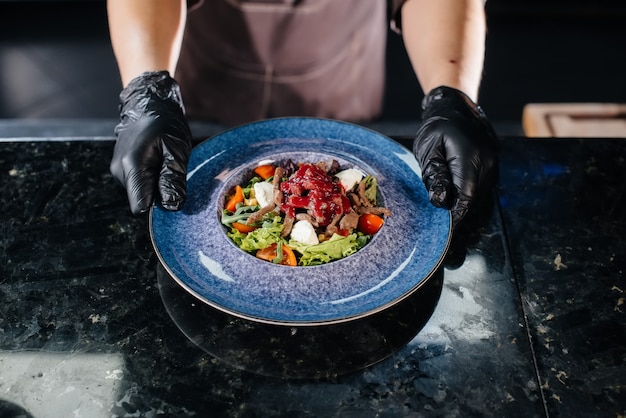This professionally taken photograph features a striking display of an elegantly prepared culinary dish situated on a black and white marbled granite countertop. The focal point is a large, aesthetically unique serving platter that blurs the line between a bowl and plate, adorned with a blue and purple marble texture. The plate itself holds a vibrant assortment of food: red and white elements, possibly cherry tomatoes and cauliflower, green leafy vegetables that might be broccoli, orange slices likely to be carrots, and a central piece of meat topped with a rich red sauce, potentially resembling meatloaf with barbecue sauce. The intricately arranged dish highlights a sophisticated mix of colors and textures, suggesting a high level of culinary artistry.

Behind the counter, partially out of focus, stands a person wearing a brown apron. Only their forearms, hands clad in black nitrile gloves, and a hint of their abdomen are visible, emphasizing their role in placing or presenting the dish. The composition hints at a professional setting, possibly the polished environment of an upscale restaurant. The photograph's horizontal alignment and inclusion of ambient details, such as the faint glimpse of gray tiles in the upper left corner, contribute to a well-balanced, visually appealing image that captures a moment of culinary finesse.